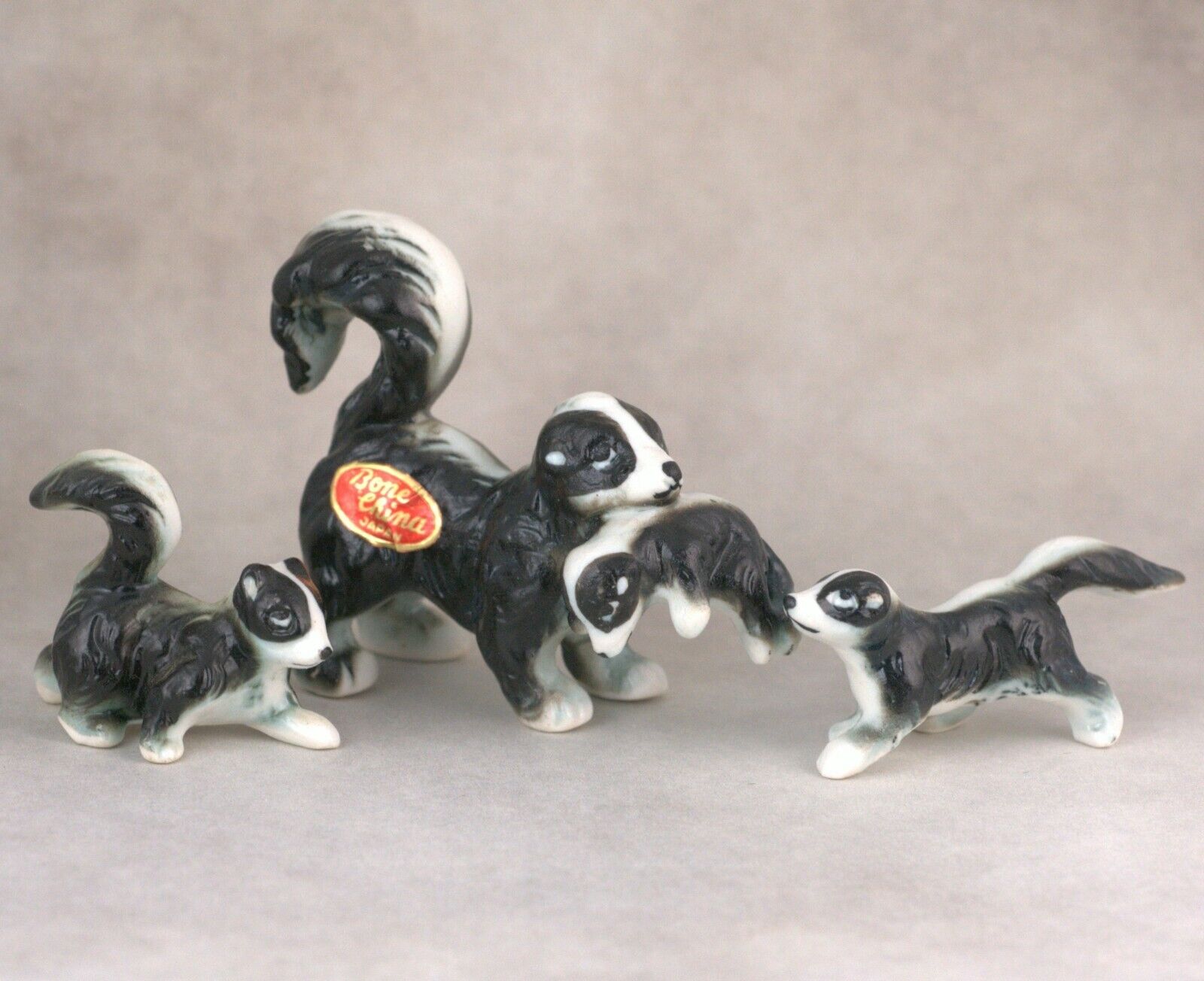This image showcases a charming family of bone china skunk figurines arranged against a light background that varies in description but is generally considered light beige or purple. The primary subject is a mother skunk distinguished by a red sticker with gold text reading "Born China, Japan," indicating the material. The scene depicts four skunks in total: the mother is holding the tiniest skunk in her mouth, while the other two baby skunks flank her on either side. These figurines have a distinctive black and white coloration, with a white stripe extending from their noses, over their heads, down their backs, and to the tips of their curled tails. Their paws and the area under their chins are also marked with white. Set in what appears to be an artfully arranged display, these lifelike porcelain ornaments seem to be playfully posed, capturing a moment of interaction within this adorable skunk family.